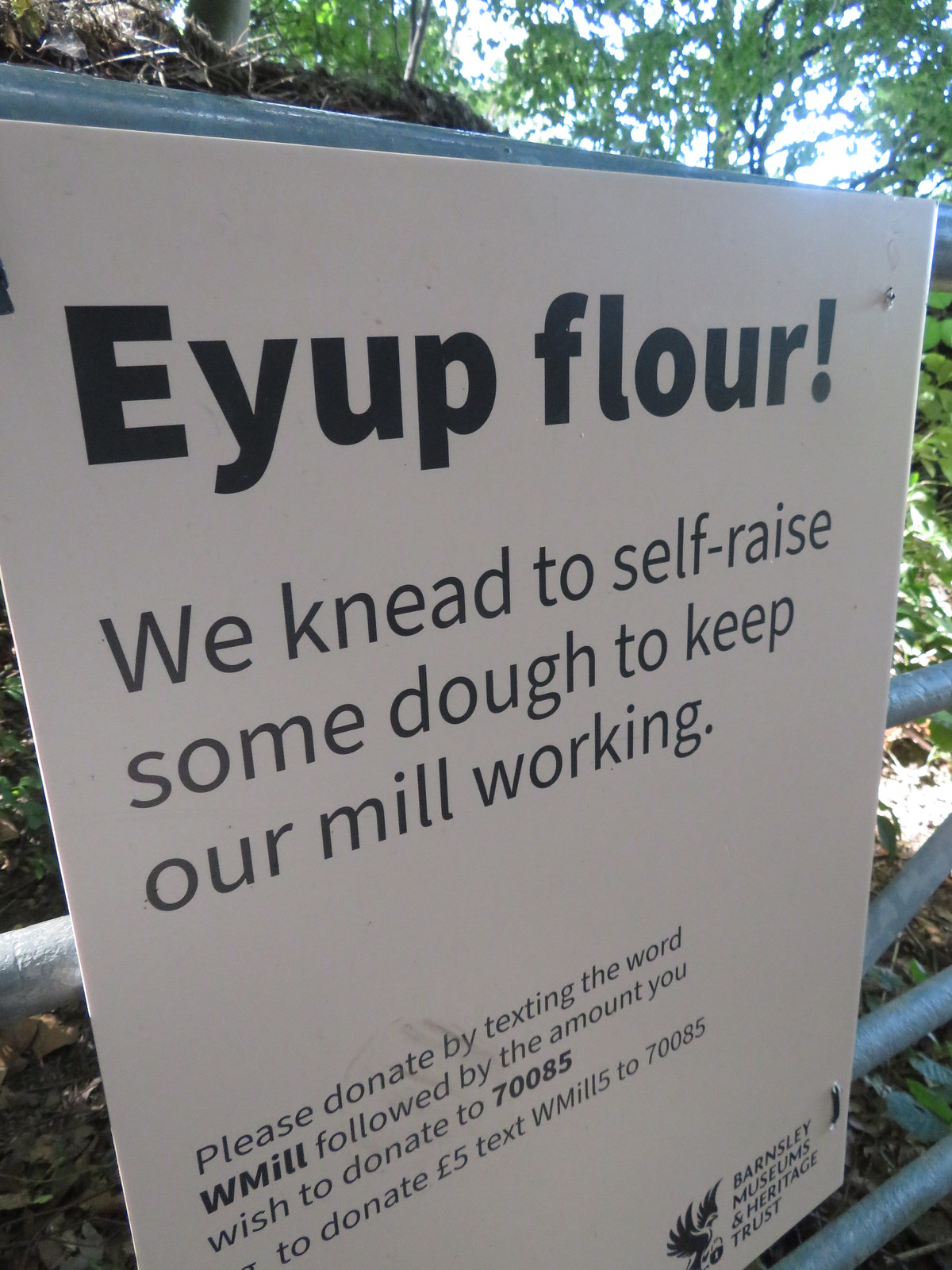This close-up photograph features a white sign posted on a metal gate, which is painted slate blue and seems to be located in a park or farm setting. The background indicates a forested area with bright sunlight filtering through green leaves, suggesting a very sunny day. The sign, measuring approximately a foot high by a foot wide, prominently displays text in black letters. At the top, in bold and large font, it reads "EUP FLOUR!" Below that, the slightly smaller text states, "We need (with 'knead' spelled as a playful pun) to self-raise some dough to keep our mill working." Further instructions are given for donations: "Please donate by texting the word WMILL followed by the amount you wish to donate to 70085. To donate five pounds, text WMILL5 to 70085." On the lower right corner of the sign, there is a logo that resembles a person flying with wings and text indicating the affiliation with Barnsley Museum of Heritage and Trust.